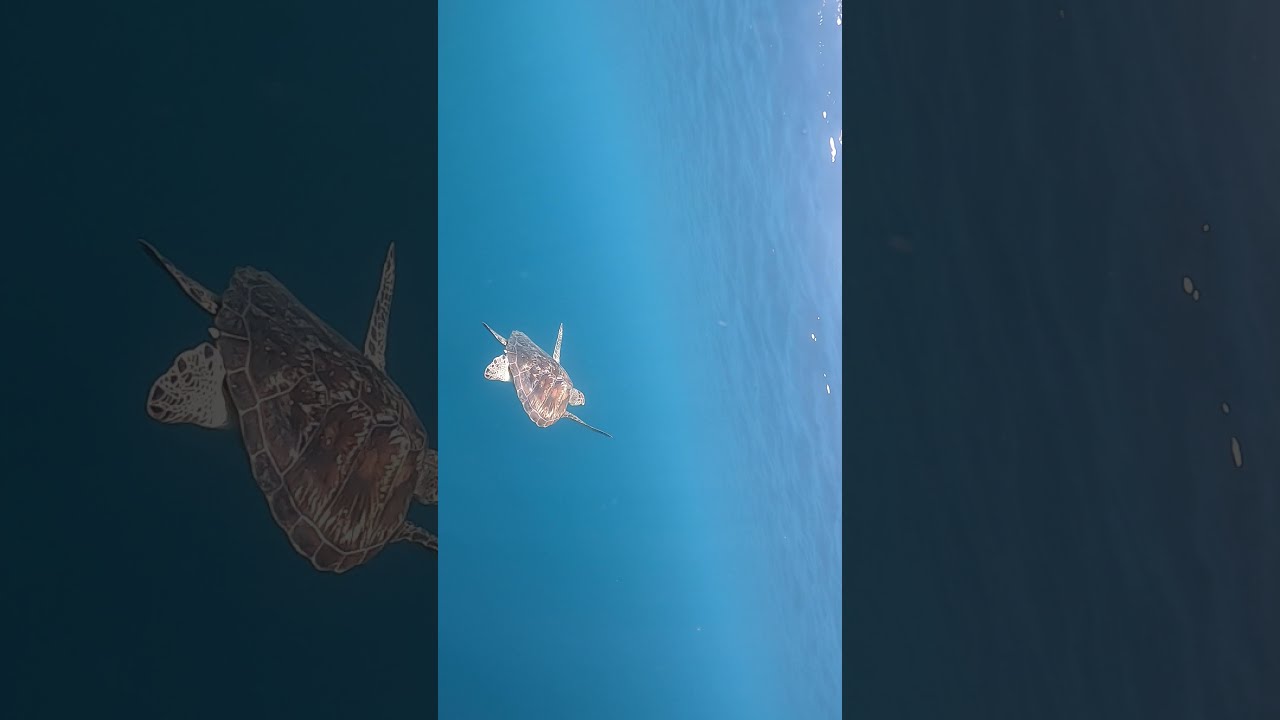In this visually striking, horizontally rectangular, full-color photograph, we see an intricately detailed underwater scene captured during daylight hours. The image is divided into three vertically rectangular panels, with the left and right panels being slightly larger and darker, serving as blown-up segments of the central panel. The centerpiece features a majestic sea turtle swimming gracefully through crystal-clear, richly blue water. The turtle, predominantly brown with a spotted texture, is oriented near the surface, where the water's ripples and sun-dappled textures are vividly visible. The sea turtle has a tail and three visible flippers, while one back flipper is out of sight. The scene is serene and undisturbed, showcasing the turtle alone in its aquatic habitat without any other creatures or objects, emphasizing its solitary journey through the vast ocean.